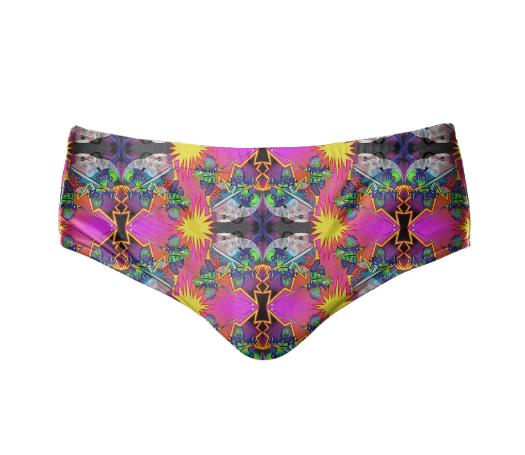This image features a colorful pair of underwear, possibly female or a men's speedo, set against a white background. The design is intricate and vibrant, showcasing an array of geometric and abstract patterns. Prominent elements include bursts of yellow that resemble explosions or suns, accompanied by vivid pink shapes. There are numerous black rectangles leading towards the middle, accented by black diamonds on their edges. Additionally, there are small, cylindrical shapes evocative of keyholes, but with an abstract twist. The background is a complex blend of tie-dye-like green, purple, and blue colors, giving it a psychedelic feel. Grey and white circular shapes add further complexity to the design, making it appear almost cluttered or busy in some areas. Floating green alien-like figures add a whimsical touch to the overall chaotic yet fascinating pattern.